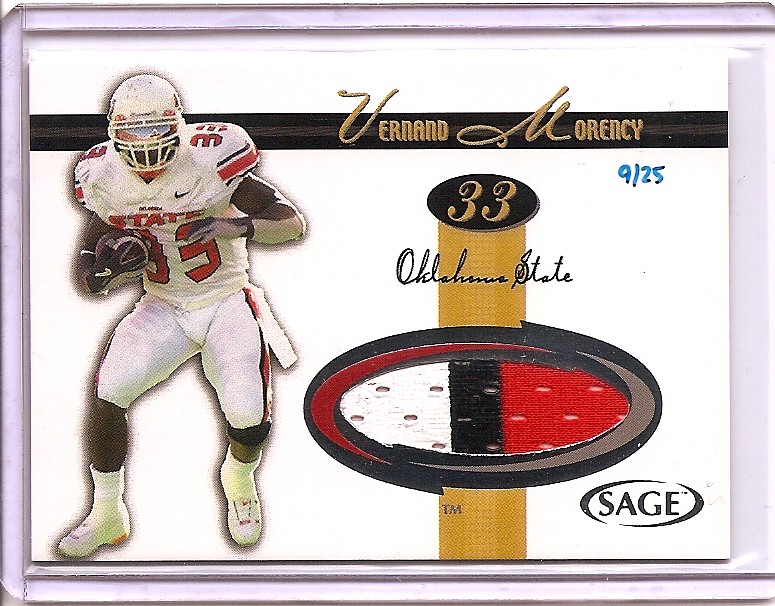A detailed player trading card for college displayed on a white background with a silver frame. The focal point is Vernard Morency, an Oklahoma State football player, depicted in his white uniform adorned with gold lettering and sporting the number 33. He is captured mid-action, carrying a football in his left hand. At the bottom of the card, the distinctive Oklahoma State logo stands proudly. The card bears the word "Sage," adding to its authenticity. Notably, "9-25" is handwritten in blue marker, though no year is specified.